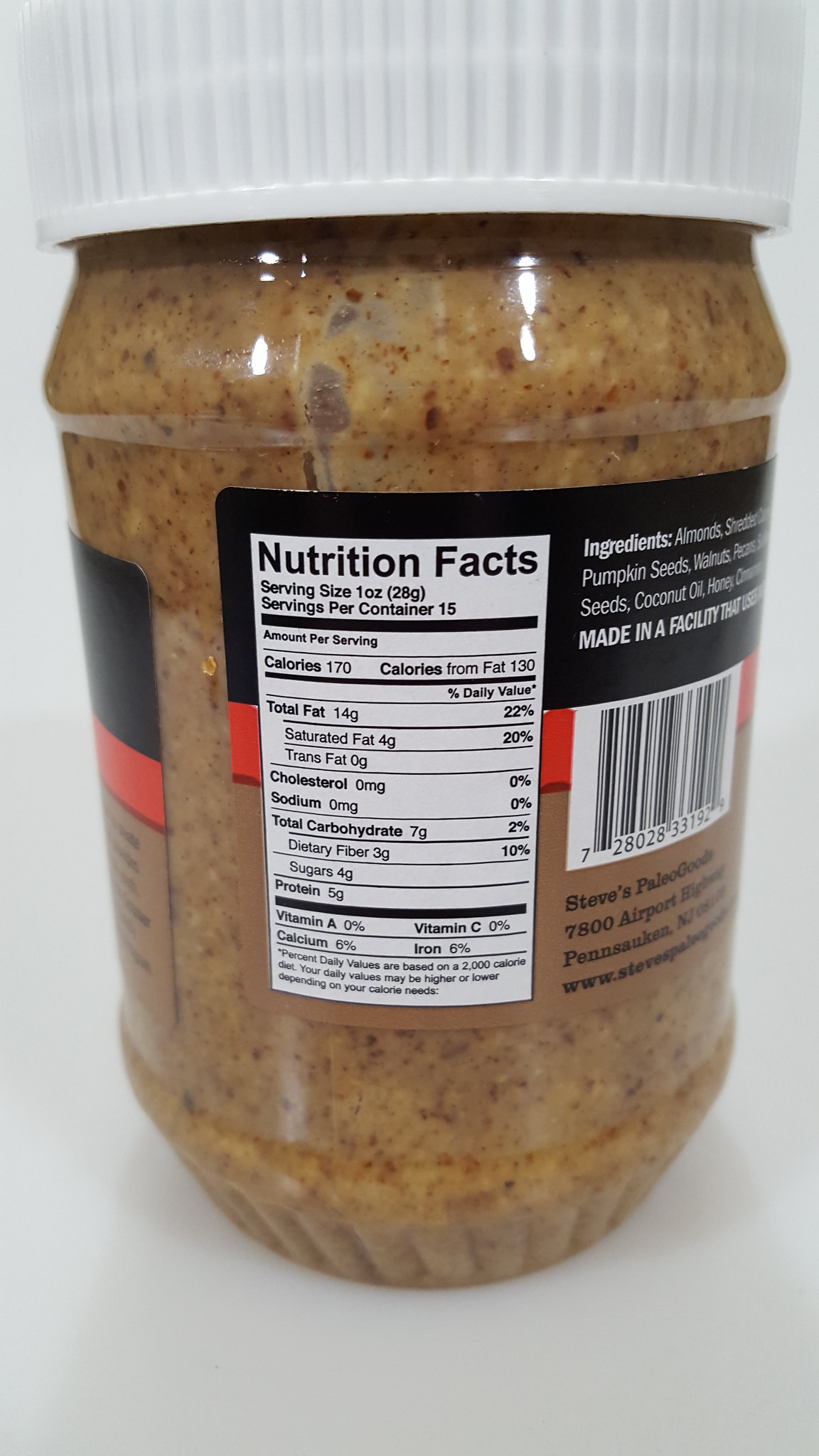### Descriptive Caption:

This close-up photograph captures a part of a label on a jar of food, centrally positioned against a white background. The jar features a distinctive shape, narrower at the bottom and widening towards the top, with a rounded form. The label itself is designed with a black background at the top, followed by a horizontal red line, and then transitions to a clear section. 

On the left-hand side of the label, the prominent, tall Nutrition Facts box can be seen. To its right, the upper portion of the label features white text against the black background. Below this, within a white square, lies the UPC code, showcasing black numbers at the bottom and vertical black lines extending upwards.

Beneath the UPC code, additional black text is visible. The jar is capped with a white lid that has ridges around its edge, adding texture and grip. Inside the jar, the contents appear to be a grainy peanut butter, exhibiting a brown hue interspersed with spots of darker and lighter brown, suggesting a rich, textured spread.